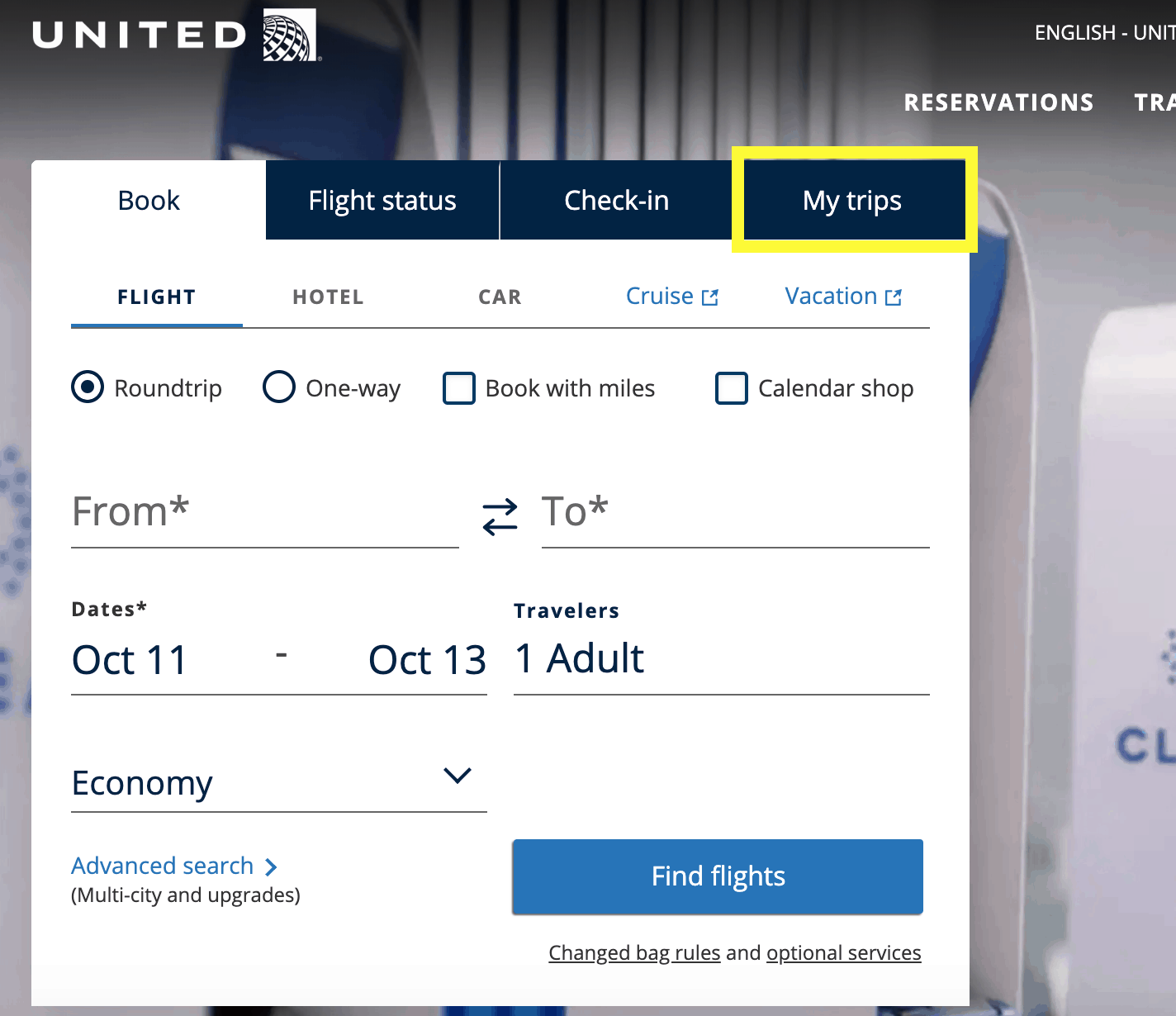---

Caption:

The image displays a United Airlines flight booking interface on an airplane, situated near the cabin divider door between regular class and first class. The interface prominently features the "United" branding in capital letters on the top left, alongside their iconic white square logo with a blue globe, partially emerging from the bottom left corner.

The booking panel includes various sections and menus: 

- The top menu showcases four tabs – "Book," "Flight Status," "Check-in," and "MyTrips" (highlighted in a yellow square). 
- Beneath the selected "Book" tab, sub-options "Flight," "Hotel," "Car," with "Cruise" and "Vacation" displayed as linked items accompanied by icons of squares with outward-pointing arrows.

Currently, the focus is on booking a flight, indicated by a blue underline. The flight search form includes:

- Two radio buttons for "Round-trip" (selected) and "One-way."
- Checkboxes for "Book with miles" and "Calendar shop."

The form fields include:

- "From" and "To" fields (marked with asterisks), presently blank.
- Date fields showing "October 11th to October 13th."
- A traveler field listing "1 adult."
- An "Economy" class selection with a dropdown arrow, all underlined.

Below these fields is a blue "Advanced Search" link and a note "(multi-city and upgrades)". To the right, a blue "Find Flights" button with white text initiates the search process. 

Further below are two important links: "Change bag rules" and "Optional services," directing users to respective information pages.

The comprehensive interface showcases United Airlines' efforts to provide a streamlined, user-friendly experience for booking flights and related travel services.

---